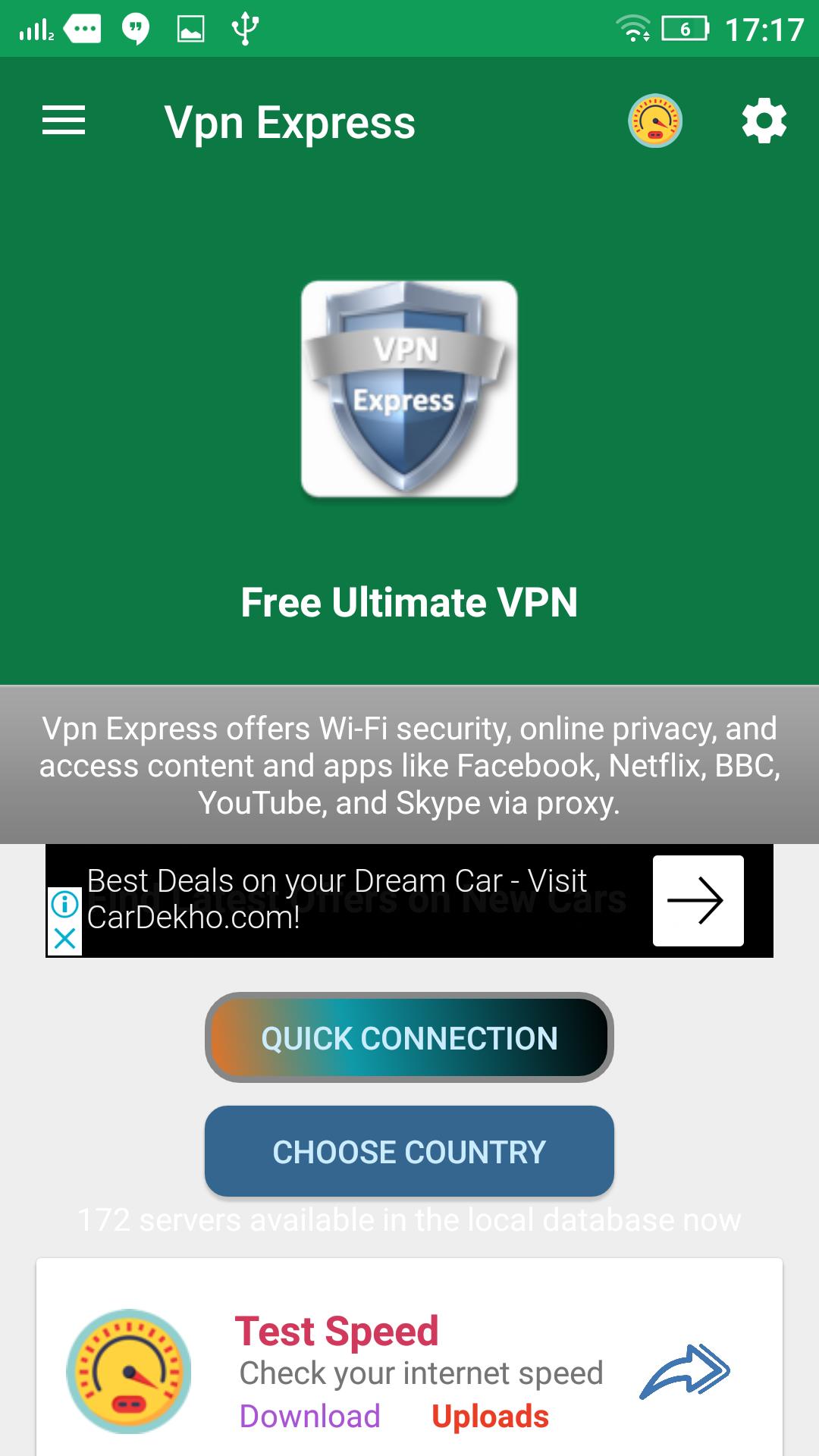A screenshot taken on a mobile phone at 17:17 military time captures the VPN Express website interface. The phone's status bar reveals a battery level at 6%, Wi-Fi connectivity with 2 bars, and several icons including a trident-like symbol, an image of a mountain range, quotation marks, an alternate battery icon, and another showing 4 bars of varying heights.

The focus is on the VPN Express, a free and ultimate VPN service. The service promises Wi-Fi security, online privacy, and access to various content and applications such as Facebook, Netflix, BBC, YouTube, and Skype through proxy servers. A clickable banner ad promoting the best deals on dream cars from cardeco.com is also visible. 

Options for quick connection and country selection are available, along with a banner for speed testing. The interface features a menu bar symbolized by three horizontal lines, the VPN Express logo, and an icon resembling a dash cam with numeric data adjacent to it and a hand pointing towards the numbers at the bottom right. There is also a settings icon, depicting tools, highlighting further configuration possibilities.